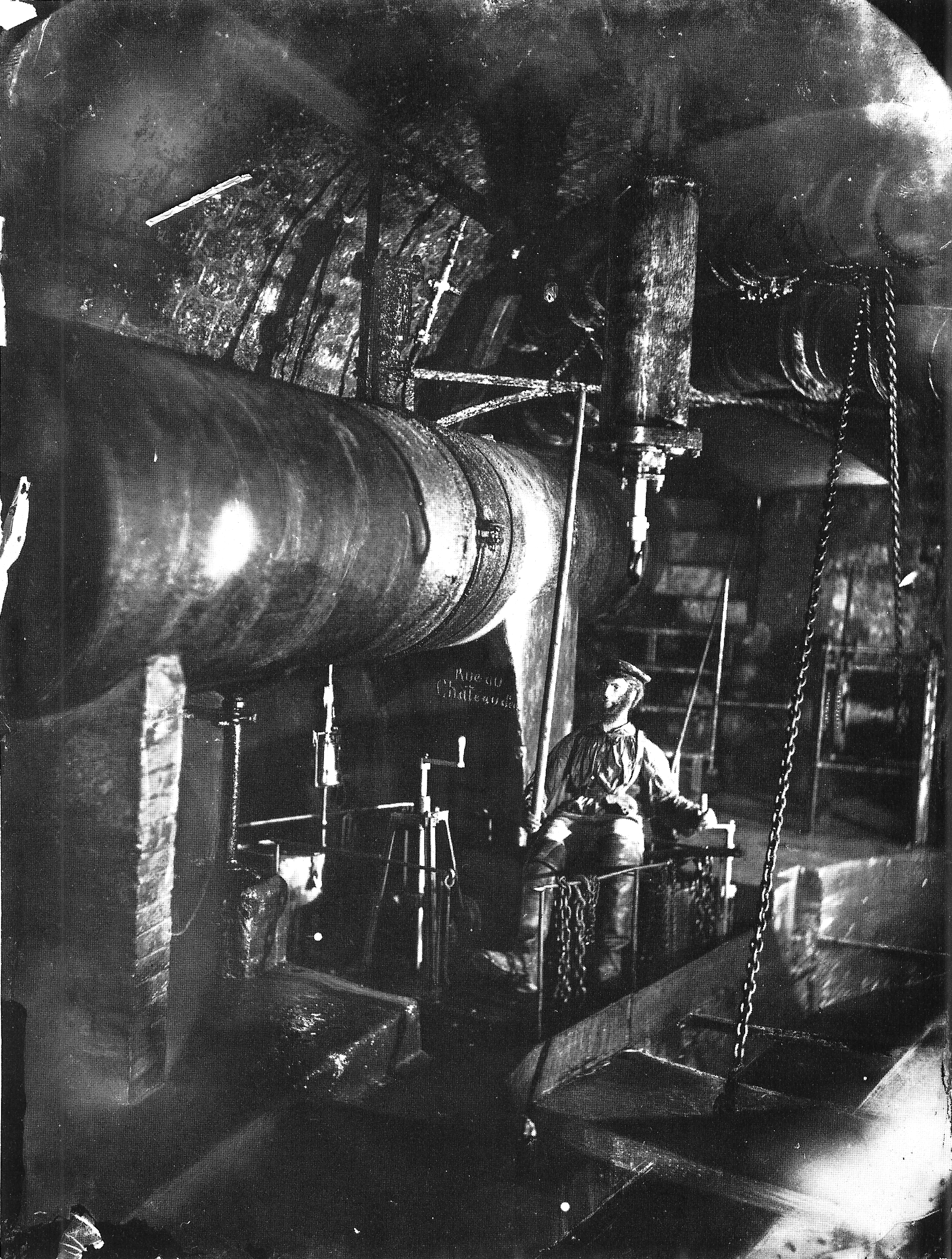This black and white photograph, presumably taken in the 1930s or earlier, depicts a detailed scene that appears to be either underground or within a factory-like setting. Dominating the left side of the frame is a large cylindrical pipe, indicative of industrial infrastructure. To the right of this pipe stands a male worker—a bearded white man sporting a beanie and clothing typical for the era, including sturdy boots and a baggy shirt, which add to the authenticity of the period captured. The worker appears to be interacting with a piece of equipment or holding a long stick-like tool in one hand, while his other hand grasps a lever, suggesting he's engaged in some form of mechanical operation. The environment is densely packed with industrial elements, including several chains hanging from the ceiling and attached to the ground, as well as other smaller devices and stands, one of which resembles a surveying tripod with a handle. The backdrop is a brick wall, adding to the industrial ambiance of the scene. The meticulous details and the apparent miniature scale of the figures create an impression of a model, yet the intricate replication of a historical industrial or steam room setting makes it visually convincing.